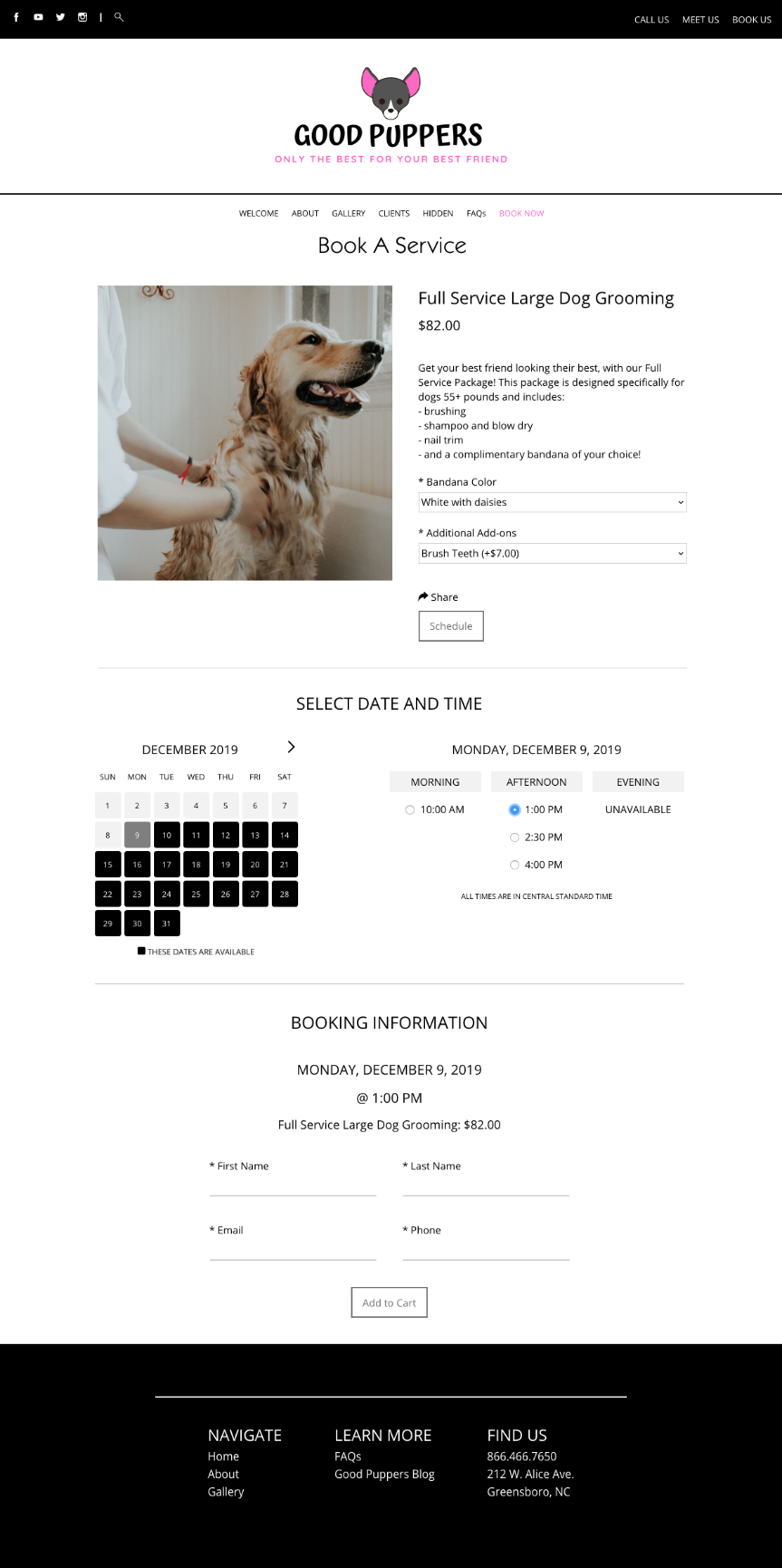This screenshot showcases a grooming service website with a well-organized layout. At the top, a black navigation bar runs across the entire width, featuring five buttons on the left and three links on the right. Beneath this bar, a logo of a black and white dog head with pink ears is prominently displayed, accompanied by the text "Good Puppers." Directly below the logo, pink text reads, "Only the best for your best friend." A black line divider follows, separating the header from the main content area.

The main content starts with seven links arranged horizontally, with the first six in black and the last one in pink. Below these links, an eye-catching headline "Book a Service" is straightforwardly positioned. On the left side, there is a warm photograph of a golden retriever enjoying a bath, while directly to the right, the service description reads "Full Service Large Dog Grooming, $82." Finally, the lower section of the screenshot features a calendar on the left side, presumably for booking appointments. The entire presentation is cohesive and visually appealing, ensuring easy navigation and a pleasant user experience.